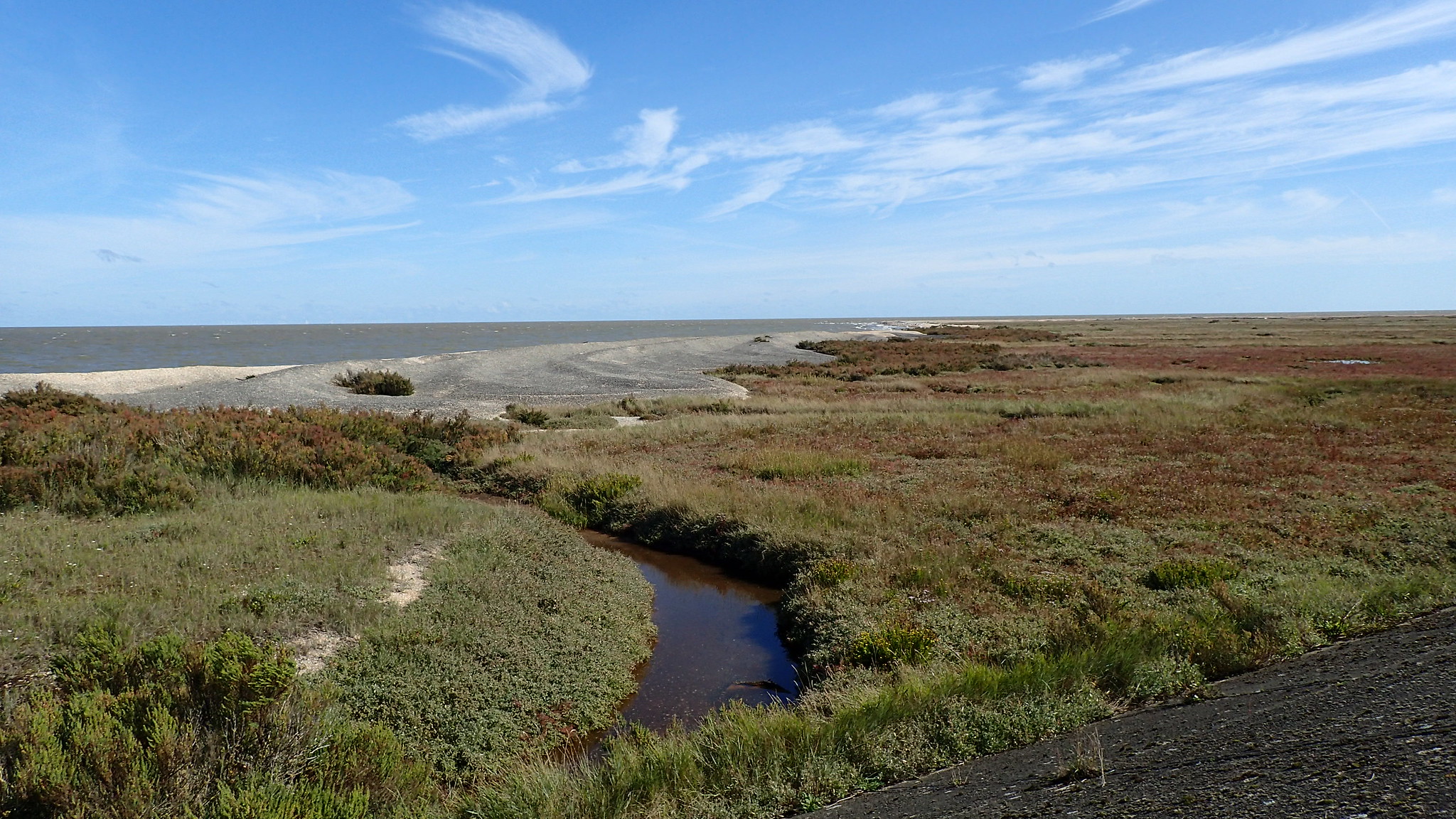This photograph captures a sprawling seascape that melds into a landscape, characterized by a sweeping wetland extending towards a large body of water, possibly the ocean or a significant lake. The foreground and mid-ground are dominated by vibrant marshland interspersed with short, marshy foliage in hues of green, brown, and occasional red. A stream meanders from the lower middle of the image, winding its way and disappearing off to the left. This stream leads towards a sandy beach area, hinting at estuarine pools filled with silt. The aforementioned pools suggest the presence of tidal influences, particularly noticeable in the upper right section. The sky above is a striking, bright blue, adorned with wispy high-flying clouds that streak across the horizon, emphasizing the clear and bright weather on the day the photograph was taken.